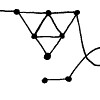In this small, intricate image, we observe a series of connected black lines forming geometrical shapes, accented by prominent black dots indicating their connections. The primary structure is an inverted triangle, with substantial black dots at each of its three vertices. Extending slightly beyond the upper-left tip of this triangle is a continuation of the line. Inside the inverted triangle, an upright triangle is neatly inscribed. From the right corner of the upright triangle, a curvilinear path descends, meeting another line that inclines from right to left. This line is marked by a small round dot, signifying a junction point where it intersects a short horizontal line. The endpoint of this short line is also marked with a dot, positioned directly below the apex of the inverted triangle.